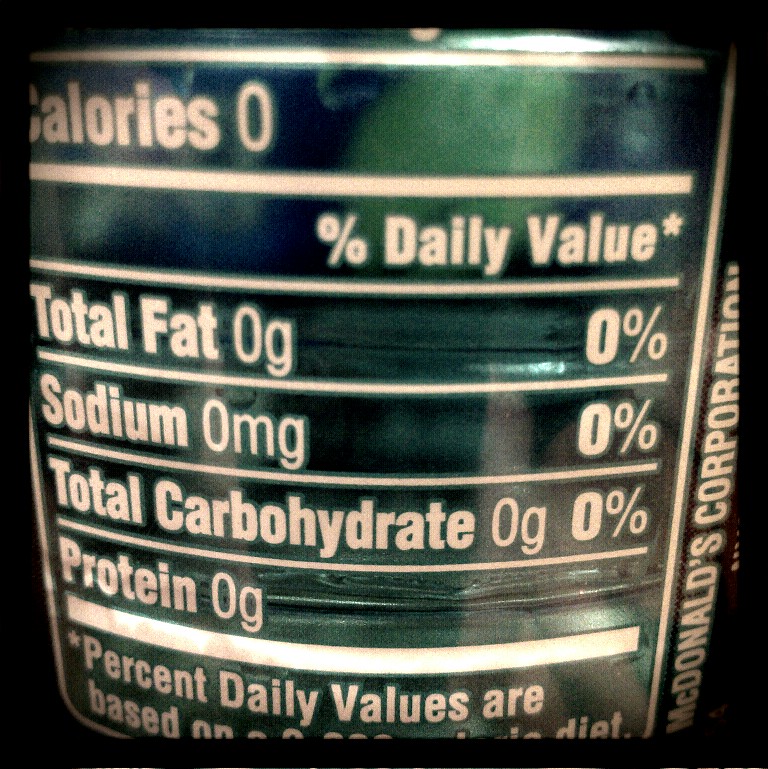This is a detailed color photograph of a green can, with the label partially visible and turned away from the viewer, making it difficult to determine its exact purpose. From the readable text on the label, displayed in white lettering, it lists the following nutritional information: zero calories, zero grams of total fat (0% daily value), zero milligrams of sodium (0% daily value), zero grams of total carbohydrates (0% daily value), and zero grams of protein. The label also notes that the percent daily values are based on a 2,000 calorie diet. Vertically printed on the right side of the label are the words "McDonald's Corporation." The photograph does not include any people, animals, plants, flowers, trees, buildings, or mechanical objects, focusing solely on the back of the green can against an uncluttered background.